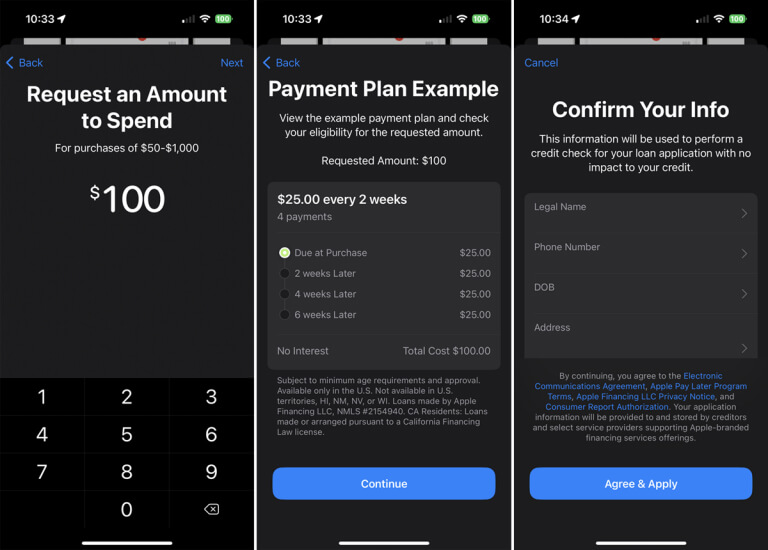This composite image consists of three screenshots from a mobile phone, each showcasing different stages of a payment request and plan selection process. 

At the top of all three images, identical black bars display the time as 10:33 with white font, alongside icons indicating active location sharing, one out of four bars of mobile signal, full Wi-Fi connectivity, and a fully charged battery at 100%.

In the first screenshot on the left, the screen has a black background with white text at the top, stating, "Request an amount to spend for purchases of $50-$1000." Directly below, in larger white font, the requested amount is shown as "$100". At the bottom of this screen, there's a numerical keypad pop-up, allowing the user to manually enter an amount.

The second screenshot in the middle introduces a pop-up menu titled "Payment Plan Example." This screen provides an overview of an example payment plan and an option to check eligibility for the requested amount of $100. Below this, a gray box details the payment breakdown: "$25 every two weeks for 4 payments." An option that has been clicked ("$25 every two weeks") is highlighted, and beneath it, additional installment options are listed: "$25 two weeks later," "$25 four weeks later," and "$25 six weeks later," all at no interest, leading to a total cost of $100. There is a "Continue" button at the bottom, presumably to proceed with the selected payment plan.